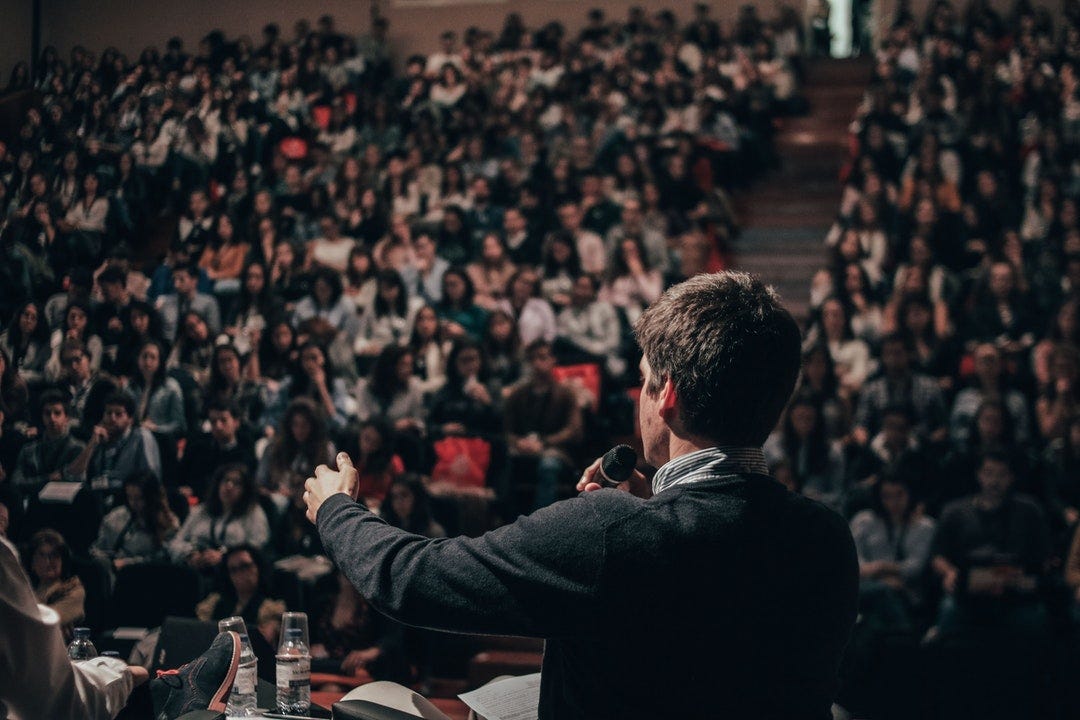This is a detailed photograph of a man giving a speech to a packed auditorium, taken from behind and slightly to the side. The man has short brown hair and is wearing a black sweater over a blue and white striped collared shirt. He holds a microphone close to his mouth with his right hand while gesturing towards the audience with his left hand. The auditorium is dimly lit, full of people seated in stadium-style seating that ascends from the stage. A staircase separates the seating into two sections. In front of the man, there is a podium that holds two bottles of water each topped with an upside-down plastic cup. In the bottom left corner of the photo, a shoe, presumably of another person sitting on the stage, is visible. This person is wearing black shoes with red trims and laces, and their leg is crossed over the other. The audience is blurred but attentive, with some individuals' hands raised. The overall setting appears to be a lecture hall or similar venue, filled to capacity.